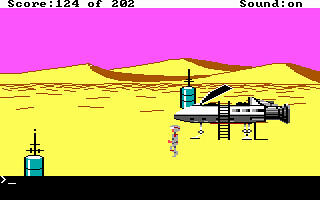This image is a screen capture from a retro-style video game, reminiscent of 80s gaming graphics, complete with a pixelated aesthetic. It depicts an alien desert planet characterized by its yellow sand dunes against a vibrant bright pink sky. At the top of the image, text reads "Score 124 of 202," followed by "Sound: On" in black letters. Dominating the scene is a white hovercraft, complete with an open cockpit, visible engines, and an extended landing gear with a ladder touching the ground.

Two turquoise barrels can be seen in the desert: one positioned near the hovercraft's right side and another at the bottom left of the image. A gray humanoid figure, possibly an alien, robot, or astronaut, adorned with red details, is walking away from the spacecraft towards the foreground. The entire image has a black border along its base, adding to its retro visual presentation.